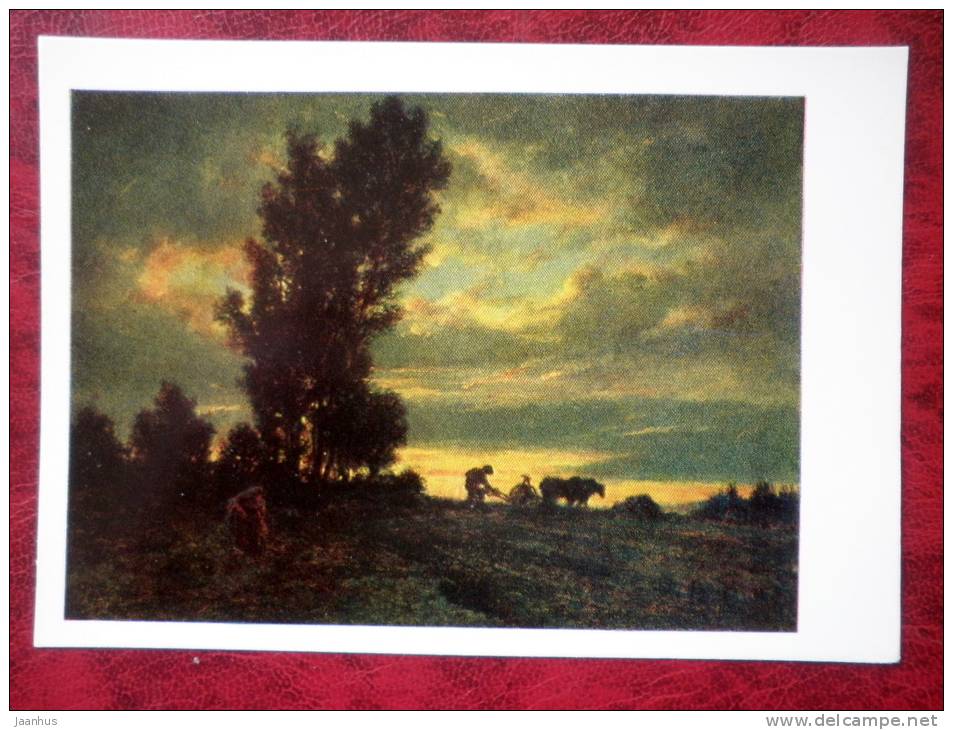The framed image, bordered in red with a white background, depicts an impressionist painting showcasing a serene, dusky outdoor setting. Dominating the left side of the scene is a large, dark tree leaning slightly to the right, its silhouette stark against a dramatic sky filled with greyish clouds tinged with hues of yellow, suggesting a recent sunset. The predominantly dark palette of the painting features deep greens, browns, and blacks. To the right of the tree, the faint silhouettes of a man and a horse (or possibly oxen) engaging in what appears to be plowing the land can be discerned, though details are obscured. The figures are shadowy and indistinct, emphasizing the overall atmosphere of the farm scene. The sky is a mix of blue and grey, with light breaking intermittently through the clouds, enhancing the tranquil yet laborious essence of the setting. This image captures the rustic beauty of a countryside scene bathed in the gentle glow of dusk.